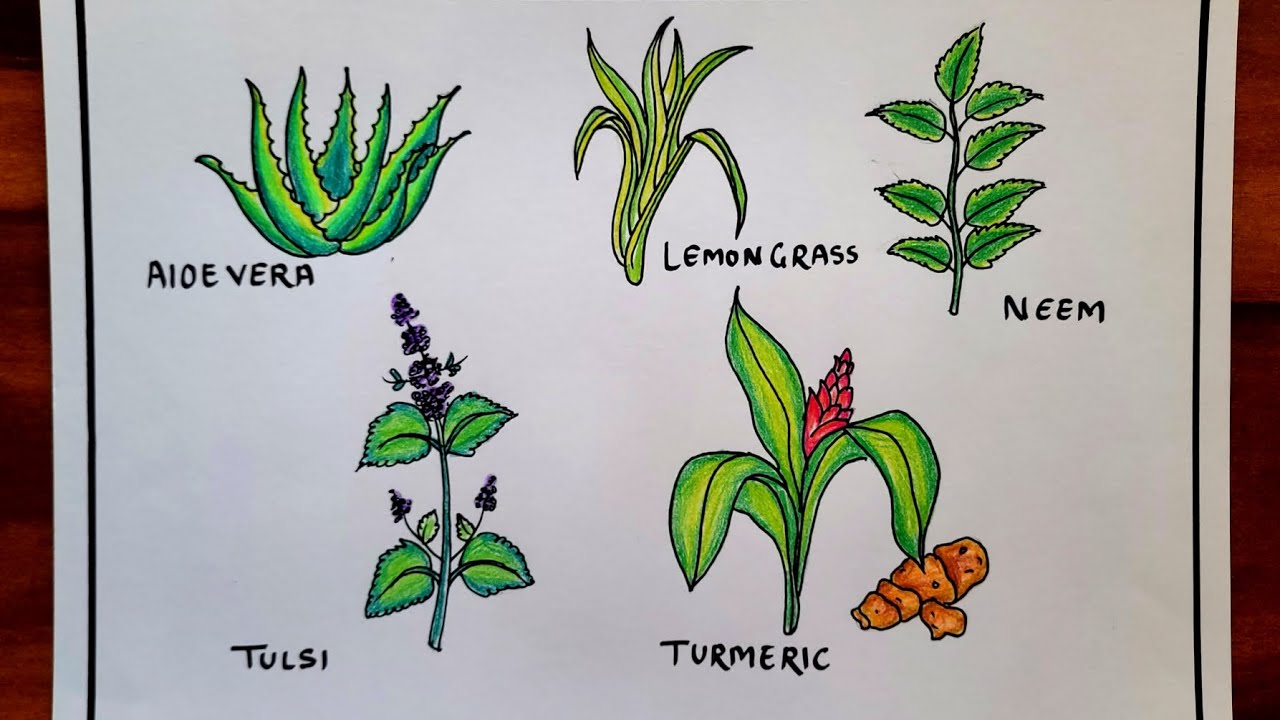In this image, there is a white piece of paper placed on a brown table, bordered by two thin black vertical strips near the edges. The paper features detailed hand-drawn illustrations of five different plants, created with a thin black marker. The plants are arranged in two rows: three at the top and two at the bottom.

At the top left, a bright green Aloe Vera plant is depicted with jagged, spiky leaves that curve outwards. Next to it is Lemongrass, portrayed with tall, wavy yellowish-green leaves resembling corn stalks without the ears. The third plant on the top right is Neem, shown as a slender, wavy stem with teardrop-shaped jagged leaves extending from smaller stems.

In the bottom row, on the left, is Tulsi. This plant features a curved stem with clusters of small purple flowers and varying sizes of teardrop-shaped leaves. To the right of Tulsi is Turmeric, identifiable by its broad, thick leaves and a distinctive red flower resembling a pinecone. At the base of the Turmeric plant, a piece of the bright orange turmeric root is drawn.

Each plant is labeled in black handwritten text beneath its illustration, enhancing the educational value and clarity of the drawing. The combination of vivid colors and fine details brings each plant to life against the stark white background.